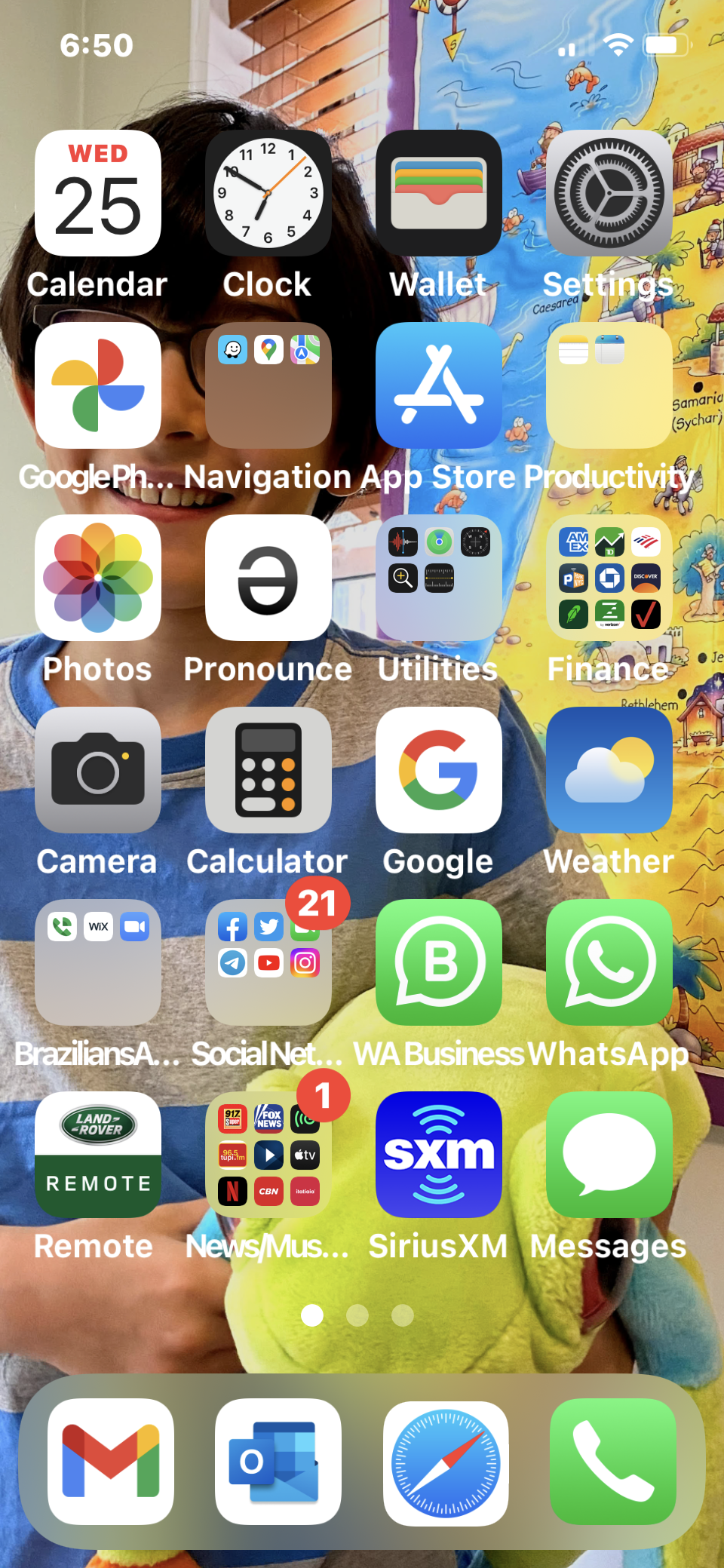This image captures the home screen of an iPhone. The background features a picture of a male wearing a blue and gray striped short-sleeve t-shirt. He is holding a small green toy frog with prominent red eyes. The man is also wearing glasses and has black hair. Behind him, there is a yellow painting with hints of blue that appears to depict a farm.

At the top of the screen, the time is displayed on the left as 6:15, while the right side shows the signal bars icon, the Wi-Fi icon, and the battery icon. The home screen is organized into several app icons arranged in rows, with four icons per row.

The first row includes:
1. Calendar app, displaying "Wednesday, 25" with "25" in black and the rest in red and white.
2. Clock app, featuring a black clock face with a white center.
3. Wallet app, illustrated as a silver wallet containing colorful cards.
4. Settings app, depicted with a gear icon.

The subsequent rows contain various apps:
- Google Photos, symbolized by a colorful pinwheel icon.
- Navigation apps for organization and productivity.
- App Store, navigation, photos, pronunciation tools, calculator, WhatsApp, and WhatsApp Business.

At the bottom dock of the screen, the primary app icons include:
- Gmail, represented by the classic Gmail envelope icon.
- Outlook, with its envelope and calendar icon.
- Safari browser icon.
- Phone call icon.